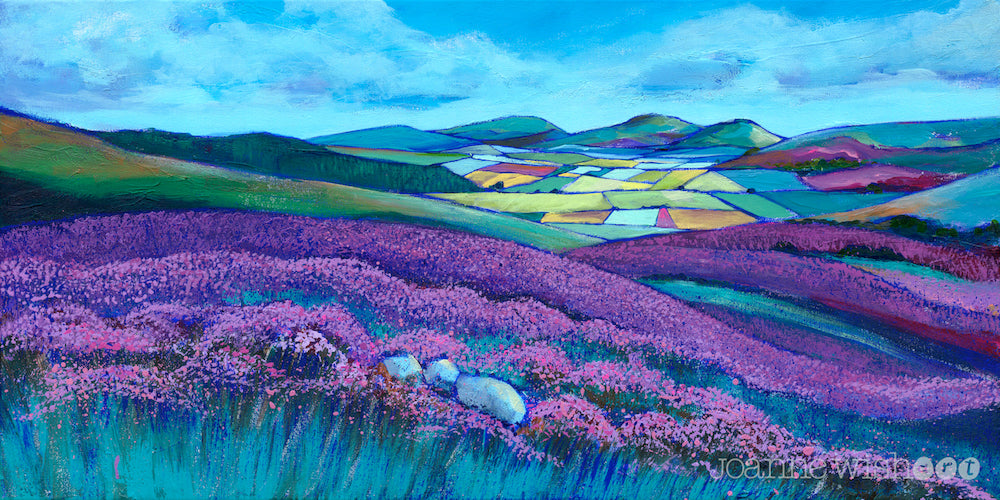This vibrant and detailed digital art piece by Joanne Wish captures a captivating landscape of rolling hills and distant mountains. The scene begins with the foreground adorned with low-lying purple flowers set against light blue grass, transitioning into a mosaic of green, orange, and muted hues that resemble stained glass. Patches of purple, yellow, and green dot the terrain, leading the eye towards the distant blue and green mountains. The sky above is a brilliant blue, punctuated with splashes of abstract purple, adding to the image's enchanting quality. In the bottom right-hand corner, the artist's name, Joanne Wish, is displayed in a transparent gray alongside small icons, possibly indicating her social media handles. This richly colored, almost horizontal piece is characterized by its beautiful and bright color palette, making it an ideal candidate for wall art.